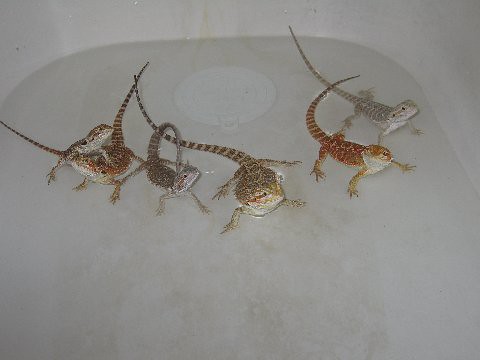The image showcases six geckos or lizards in a white bathtub partially filled with water, enough to keep their lower bodies submerged while their heads and upper torsos remain above the surface. The lighting is poor, making details somewhat harder to discern. The tub appears slightly dirty, with visible brown spots. On the left side, a small lizard, whose color is indistinct, is perched on the back of a larger lizard with a reddish back and white belly. From left to right, the lizards show a range of colors: the first with a reddish back, the second smaller and less clear in color, the third predominantly gray, the fourth brownish-black and the largest in the middle, the fifth mottled red, and the last one a light gray. They seem to be arranged in a roughly linear formation along the tub's bottom, with a bath stopper partially visible, indicating it is indeed a bathtub.